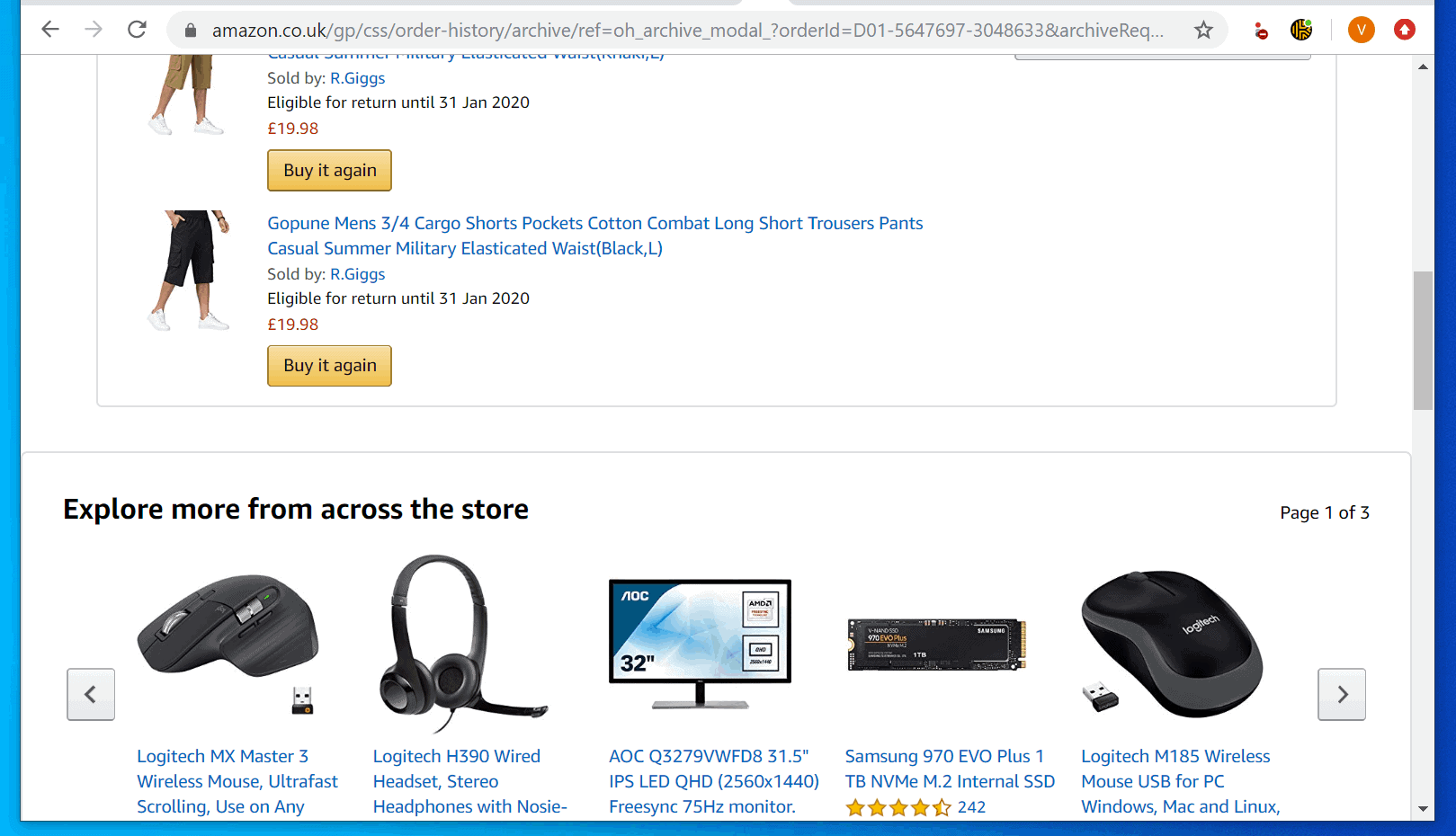The screenshot depicts an Amazon UK webpage. At the top, we see the website’s user interface elements. From left to right, there's a backward-pointing arrow icon, a reload icon, and a search bar that is displayed in gray. The search bar includes a black lock icon, indicating a secure connection, followed by the text "Amazon.co.uk." Adjacent to the web address is a star icon for adding the page to favorites, and four additional icons including a prominent orange circle with the letter "V."

Below this header section, the focus shifts to two products featured prominently on the page. The first item appears to be a pair of shorts sold by "Our Gigs," priced at $19.98, and is eligible for return until January 31st, 2020. There is also a yellow "Buy it again" button associated with this product. 

The second product is described as "Puny Men's Three-Quarter Cargo Shorts," which come with pockets and are fashioned from cotton. These combat-style, casual summer shorts feature an elastic waistband and are sold in black by "Our Gigs," with the same return eligibility date mentioned above. This item also has a yellow "Buy it again" button below its description.

Below these product listings, there is a section titled "Explore More from Across the Store," which presents a variety of recommended items based on the user's browsing history or popular searches. The entire screenshot is encapsulated within a rectangular frame that is outlined with a blue rectangle.

This detailed image provides a clear representation of the Amazon UK's web layout, specific product details, and a glimpse into the user’s shopping experience.